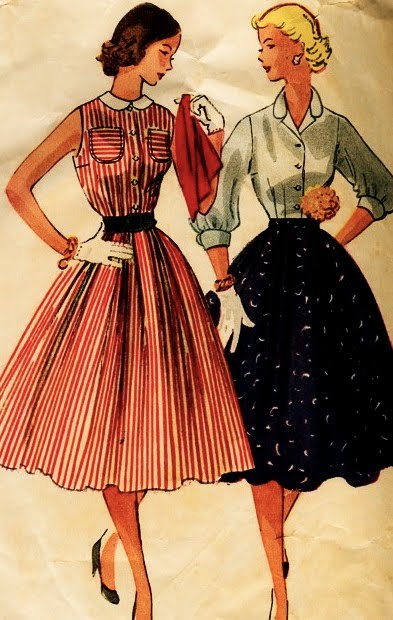Here we have a vintage illustration, reminiscent of old McCall's sewing patterns from the 40s or 50s, depicted on slightly crumpled paper which adds a nostalgic touch. The image features two women, both in cinched waist, flared knee-length skirts. 

The woman on the left has short brown hair and orangey-brown skin. She is dressed in a sleeveless dress with vertical red and white stripes, contrasting with horizontal stripes on the pockets. The dress has a white collar, black belt, and she is accessorized with white gloves, gold or orange wrist accessories, black pumps, and a white hanky in one hand. 

Next to her stands a woman with short blonde hair. She wears a light gray button-up blouse with three shades of gray and a poofy blue skirt adorned with white specks. Her ensemble is completed with a pink and black corsage at the waist and black shoes. Both women are looking at each other, capturing a moment of vintage elegance.